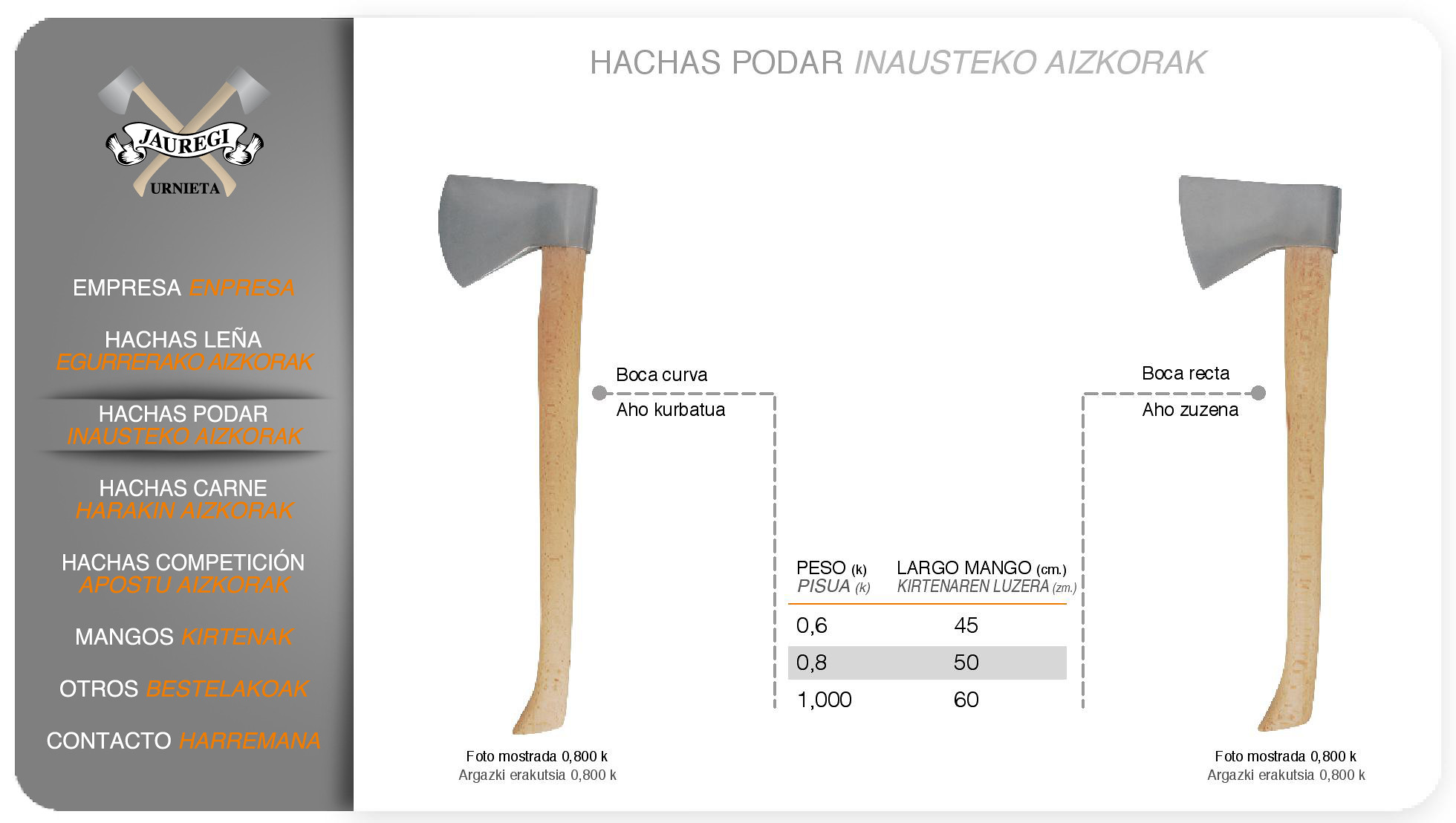The image depicts a website screenshot showcasing two crossing hand axes with grey blades and light brown wooden handles, forming an 'X' against the background. A white banner with red letters spells out "Jauregui" at the intersection of the axes. The left side of the image features a grey vertical strip displaying various features of the axes and their uses, written in multiple languages including Spanish. Terms like "empresa" (business), “hachas leña” (woodcutting axes), "hachas podar" (pruning axes), and "otros" (others) are highlighted in white and orange font. Detailed measurements and weights for each axe are indicated by dotted lines pointing towards the middle of the handles. There is a sidebar menu containing the company's logo at the top and links to different product categories such as "carne" (meat) and "competición" (competition). Light grey lettering overlays the white sections, further detailing the specifications of the axes.